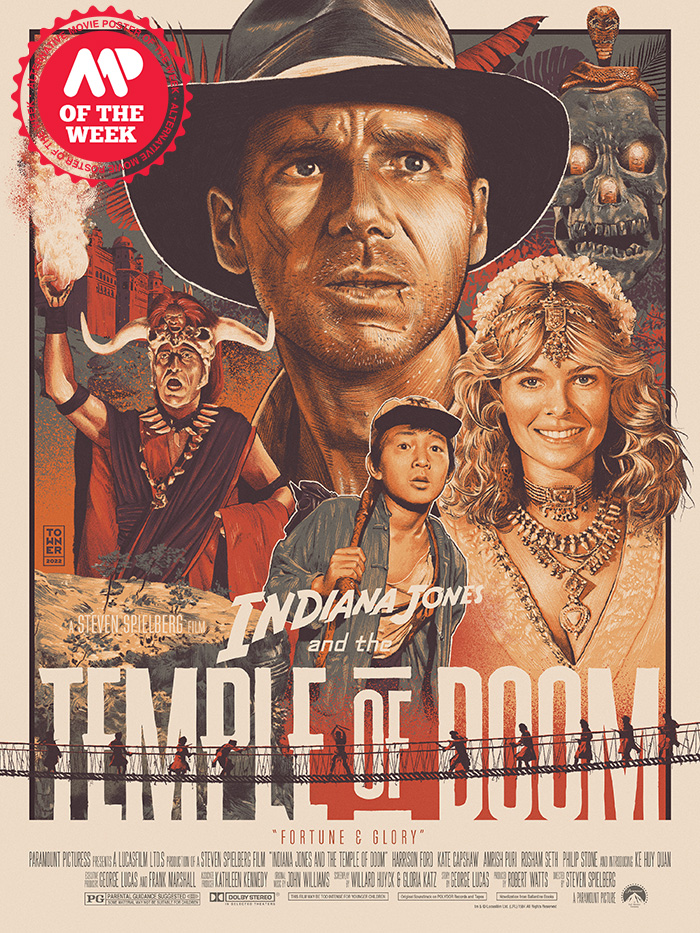This vibrant movie poster for the 1984 film "Indiana Jones and the Temple of Doom," directed by Steven Spielberg, features Harrison Ford prominently in the center as the daring archaeologist Indiana Jones, wearing his iconic black cowboy hat. Surrounding him are key characters: on the left is the villain adorned with a menacing horned headdress and a brown sash, while to the right stands Indy’s lover, a smiling blonde woman with flowing shoulder-length hair, adorned with numerous necklaces and a golden shirt. Below them, the young Asian sidekick, wearing a blue open-front shirt and a baseball cap, accompanies Indiana Jones. The dramatic scene depicted on the hanging bridge underscores the film’s adventurous spirit, with Indiana Jones caught between his pursuers. At the top left, a red circle with white letters declares "Movie of the Week: AP of the week," and centered in white font is the title, "Indiana Jones and the Temple of Doom." The lower section of the poster includes additional credits, cast names, and the film's rating, encapsulating the essence and excitement of this cinematic classic. The slogan "Fortune and Glory" hints at the thrilling escapades that await.